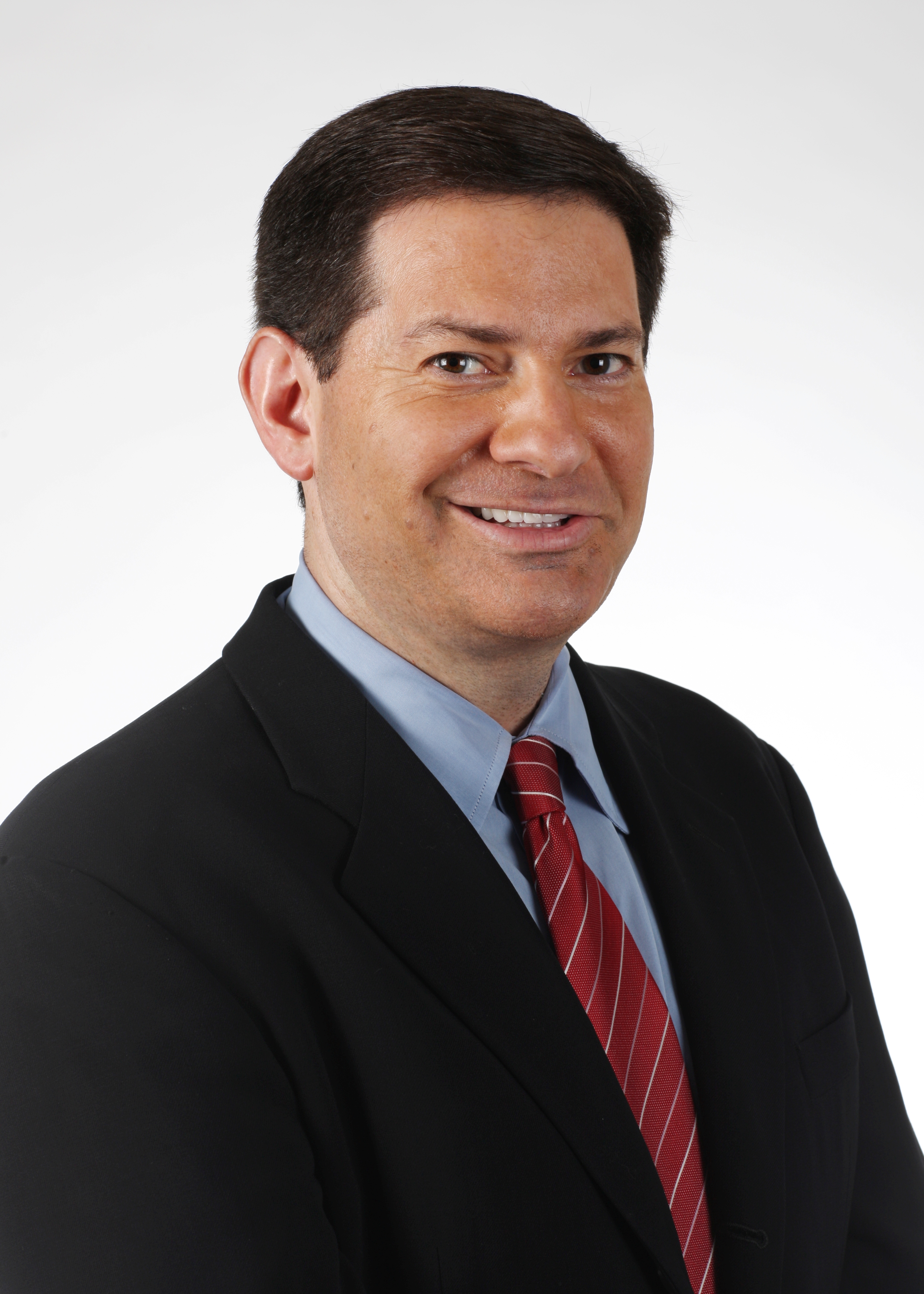In this portrait image, we see a professionally dressed man who appears to be a politician or businessman, once known as a news commentator on a morning show. He is clad in a black suit jacket, a blue collared shirt, and a distinctive red tie with silver diagonal stripes. The man has short brown hair, brown eyes, and is clean-shaven, showcasing a well-groomed appearance. He is giving the camera a smile that could be interpreted as either content or slightly forced, perhaps indicative of the personal controversies that led to his abrupt exit from the public eye due to sexual harassment allegations. The backdrop is a plain white or gray, focusing all attention on the subject himself, who stands tall and poised.